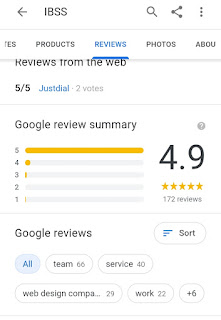This screenshot captures a section of a company's review page on Google. At the top of the screen, there is a gray left arrow. Next to it, in white capital letters, is the acronym "IBSS." To the far right, there is a magnifying glass icon for search, followed by a share icon consisting of three dots connected by two lines, and a settings menu represented by three vertical dots.

Below this header is a set of tabs: "Products," "Reviews," "Photos," and "About." The "Reviews" tab is currently selected and highlighted in blue. The section beneath the tabs reads "Reviews from the web," featuring a "5 out of 5" rating from "JustDial" based on two votes.

Following this, there's a "Google review summary" with an overall rating of 4.9 out of 5 stars. The graphic shows five yellow stars based on 172 reviews, the majority of which are 5-star ratings. There are also a few 4-star and 3-star ratings, with very few 1-star ratings.

Further down, the "Google reviews" section has a sorting option with various categories: "All" with 66 reviews, "Team" with 40 reviews, "Service" with 29 reviews, "Web Design" with 22 reviews, and a "+6" option for additional categories.